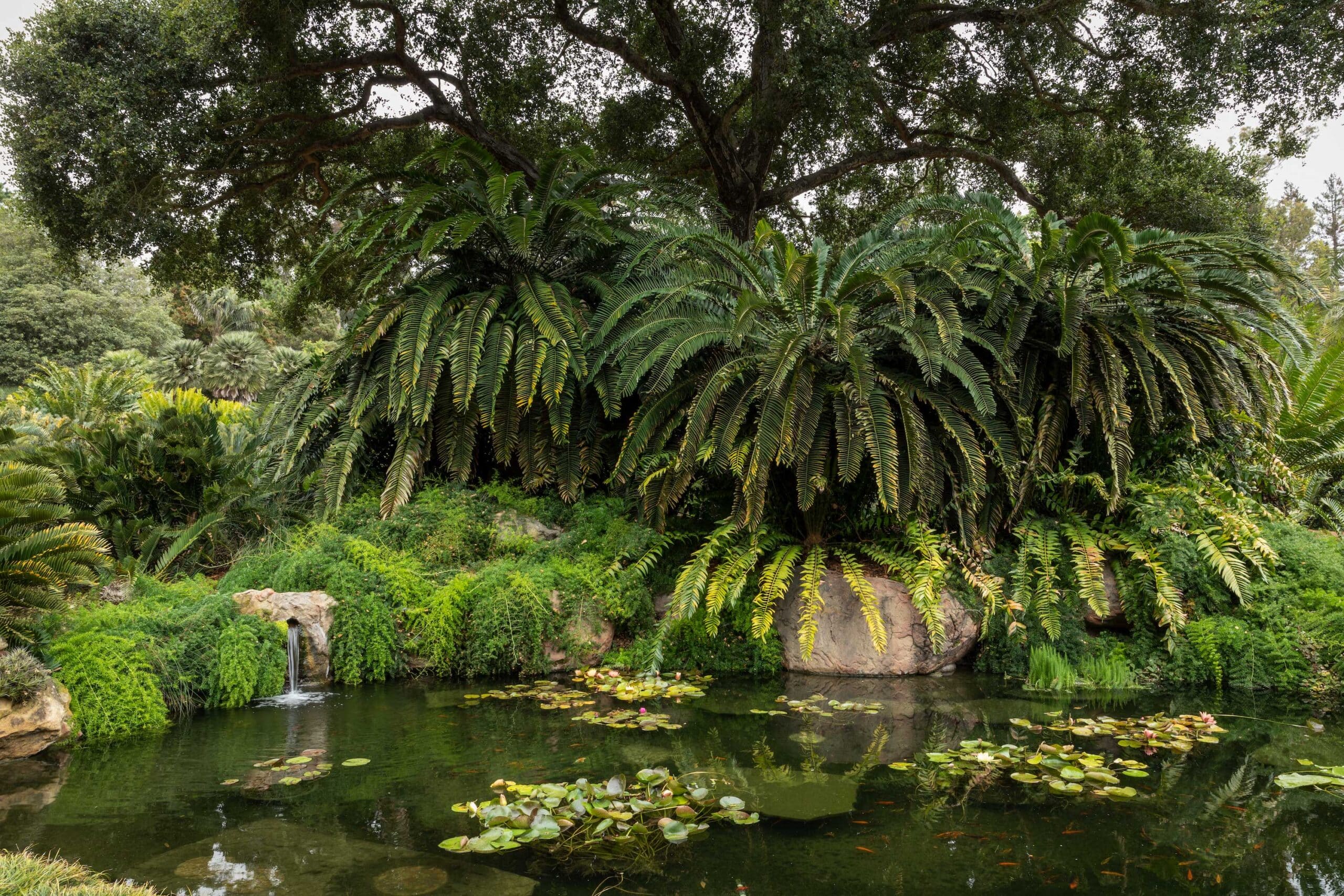This image depicts a serene, lush garden featuring a small, somewhat murky pond with green moss and floating lily pads. The water is shallow and see-through, revealing goldfish and submerged rocks on the left side. A pipe on the left bank drips water into the pond, contributing to a trickling stream. Surrounding the pond are dark gray and light gray boulders, along with a dense variety of plant life. You'll see an array of ferns, from dark green to lighter, almost yellowish shades, mingling with tropical palm trees and other greenery. A large tree with sprawling, heavily-leaved branches stands prominently in the background, creating a canopy over the area, while the sky appears white and cloudy, suggesting an overcast day. The combination of these elements makes for a secluded, vibrant, and tranquil garden scene.